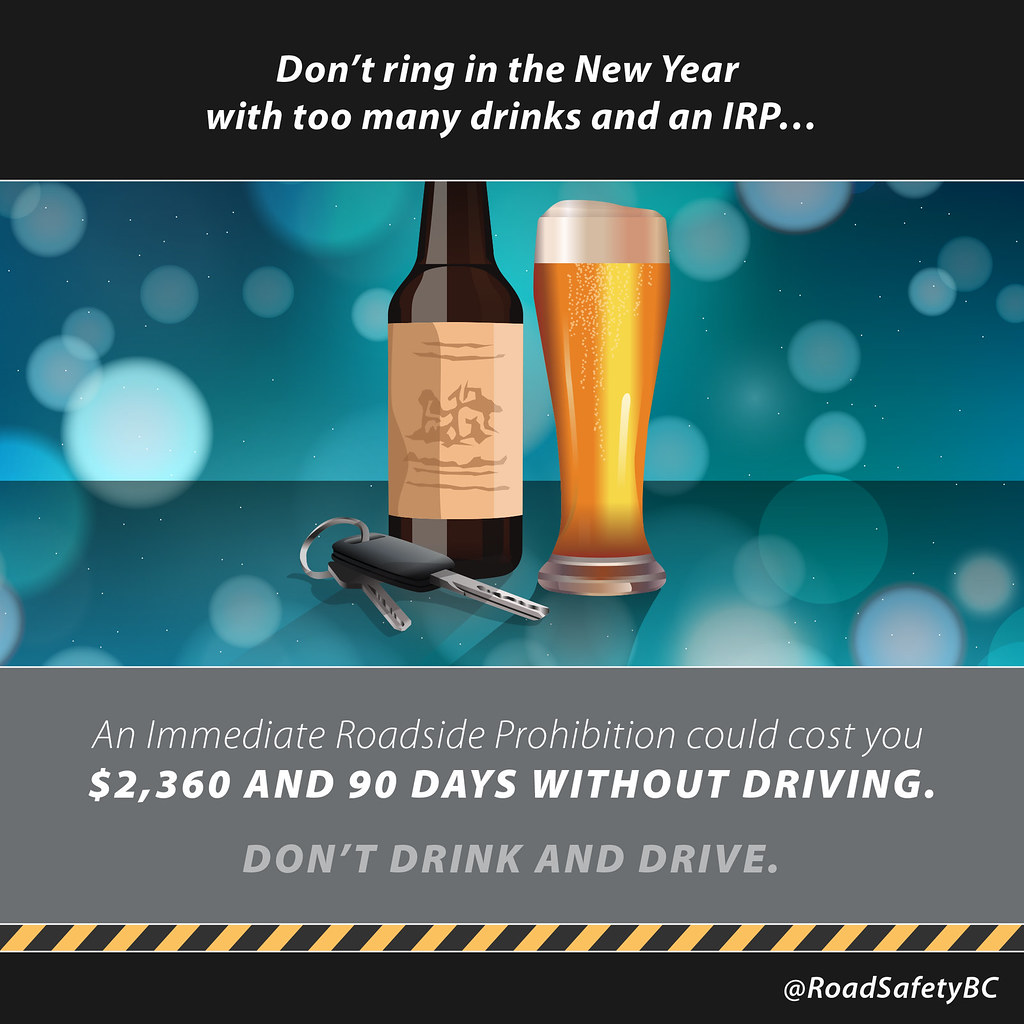This image is a digital public service announcement poster designed to raise awareness about the dangers of drinking and driving, especially during the New Year celebrations. At the very top, there is a black bar with white text that reads, "Don't ring in the new year with too many drinks and an IRP...". Below this text, the central image features a wine glass on the left and a tall glass of beer on the right, next to a set of car keys placed on a dark blue, possibly glass tabletop. The background has a light blue hue with bokeh circles, reminiscent of blurred car lights, adding to the visual theme of caution.

In the section beneath the image, there is a gray box containing white text that states, "An immediate roadside prohibition could cost you $2,360 and 90 days without driving. Don't drink and drive." The final component of the image is a diagonal yellow and black caution tape pattern at the bottom, emphasizing the serious warning of the poster. Additionally, there's a mention of "at Road Safety BC," which indicates the organization behind the PSA.